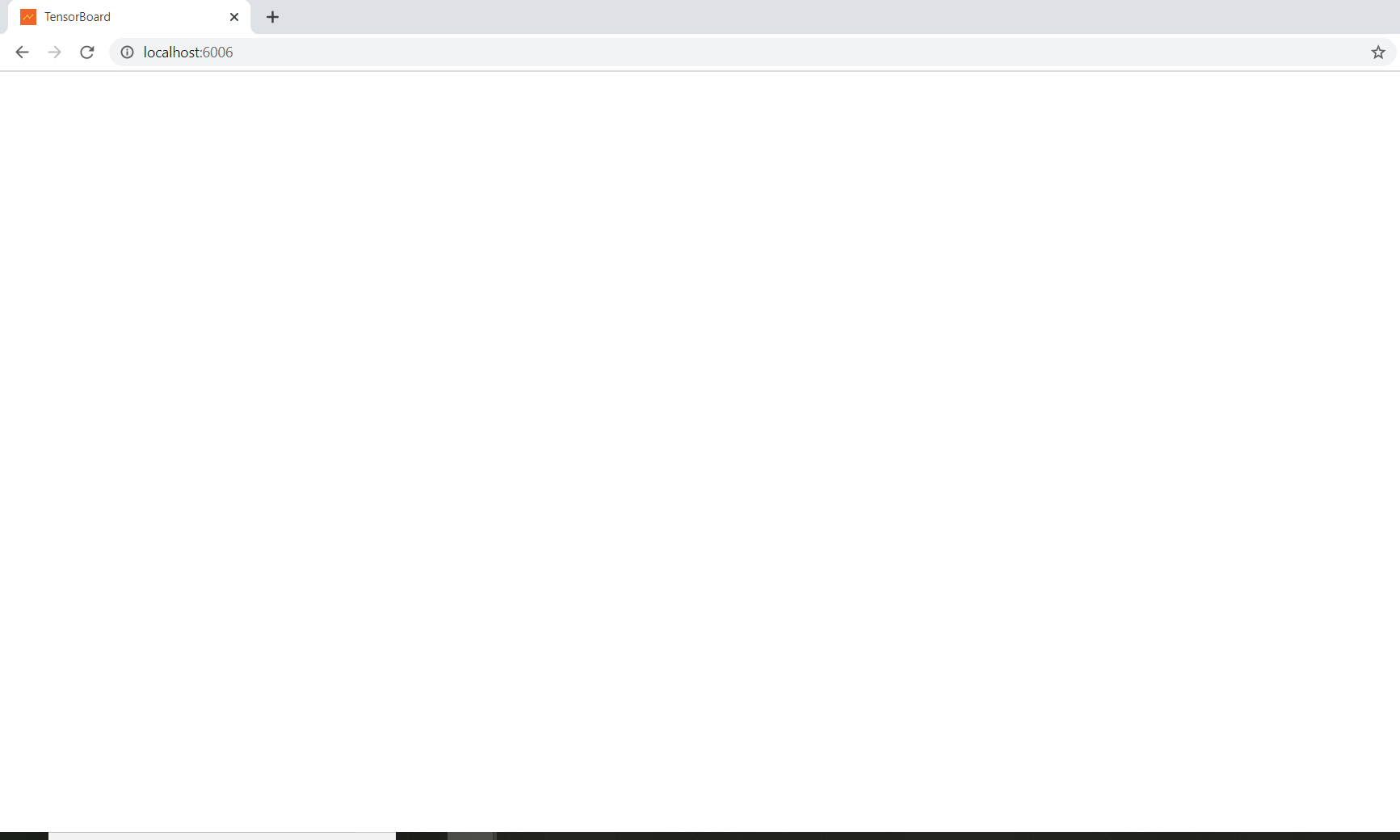In the image, we see a screenshot capturing a web browser interface displaying the TensorBoard website. The browser tab in the upper left-hand corner is labeled "TensorBoard," featuring an orange square with a distinctive white squiggle line across the center. In the address bar, the URL is "localhost:6006." To the left of the address bar, there are navigation buttons including back, forward, and refresh. On the far right of the address bar, there is an outlined star icon, which serves as the bookmark button. The webpage itself is currently blank, showing an entirely white screen. At the bottom of the screenshot, there is a thin rectangular bar that is divided into segments: the first segment is black, followed by a light gray portion, and the remainder is black again, extending to the right edge of the screen.